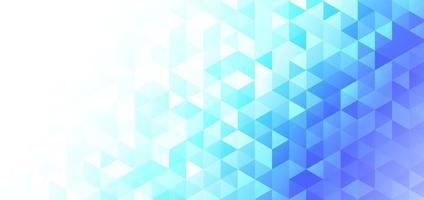This image features an abstract, computer-generated design dominated by geometric shapes, particularly triangles and three-dimensional cubes. The composition starts in the upper left with an intense white that gradually transitions to vibrant shades of teal, blue, and eventually a deep, almost purplish blue on the lower right. The color shift creates a wave-like effect, enhancing the sense of depth and three-dimensionality. The interplay of light and dark shades within the shapes adds to this depth, giving the impression of a pixelated or mosaic pattern. This modern design is versatile, making it suitable as a digital or printed background, perfect for anything from desktop wallpapers to phone screens.